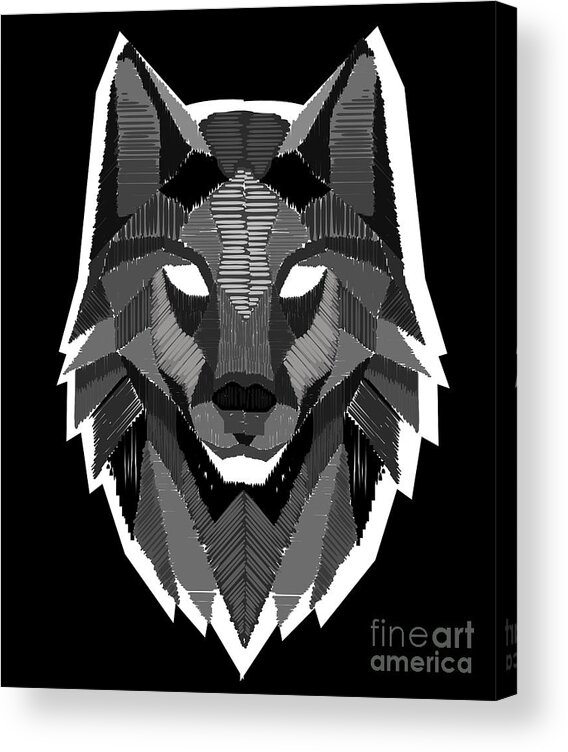This illustration depicts a majestic wolf facing directly at the viewer, characterized by its pointed ears and intense, white eyes. The artwork is rendered in a monochromatic palette of black, gray, and white, featuring intricate line work that gives the illusion of mirrored strokes, especially noticeable on the ears and the face. Despite contrasting interpretations suggesting various techniques—ranging from digital artistry imitating toothpicks to possible stitching—the consensus highlights the detailed and deliberate construction of the wolf's fur and facial structure. The silhouette of the wolf is framed by a thick white border, set against a black canvas that gives the impression of being hung on a white wall. The image bears a watermark reading "Fine Art America" in the lower right corner, with a subtle mirrored version at the canvas's edge. The deliberate use of shading and texture creates a strikingly lifelike and vivid representation of the wolf.